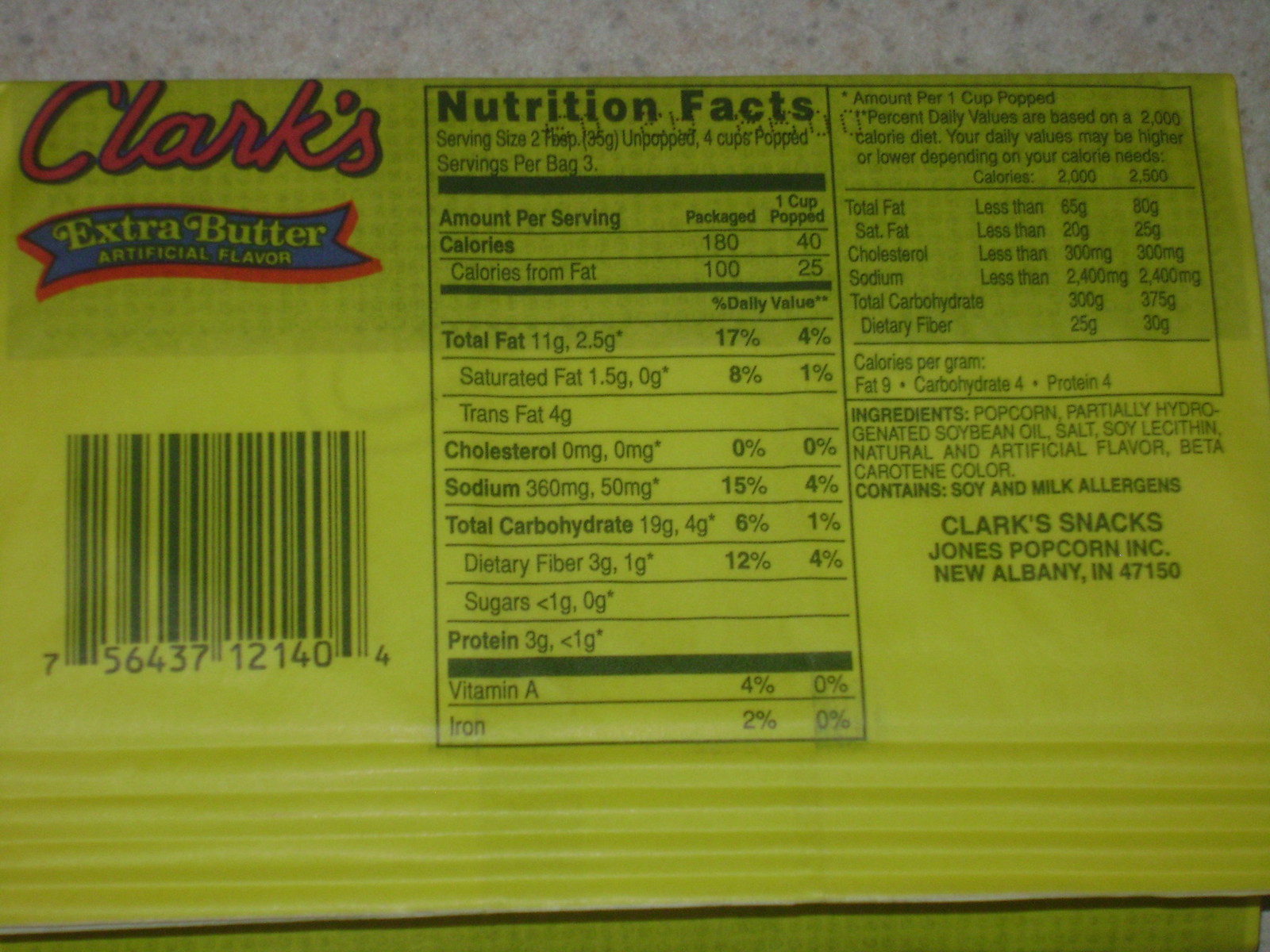A vibrant, color photograph showcasing the back of a popcorn package. The predominant yellow background accentuates the detailed information provided on the label. Positioned along the left column is the brand logo, "Clark's Extra Butter," accompanied by the text "artificial flavor" and a barcode beneath. The central column is dedicated to nutrition facts, detailing the serving size of two tablespoons (35 grams), which equals four cups when popped, with each bag containing three servings. The right column delves into specifics regarding fat, cholesterol, sodium, and additional nutritional information. Toward the bottom, the list of ingredients is provided, concluding with the manufacturer's address in New Albany, Indiana, ZIP code 47150. The meticulous arrangement of content on the package hints at the product being a bag of microwaveable popcorn.